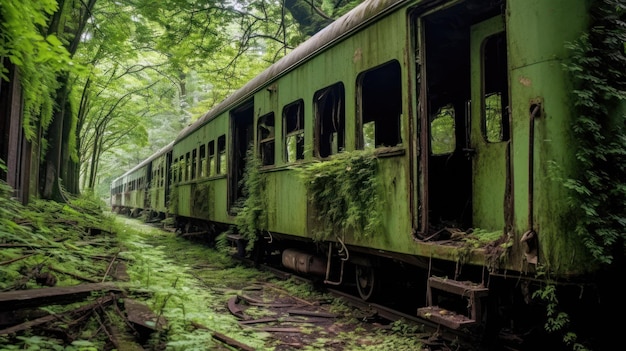This image captures an old, abandoned railroad train, seemingly forgotten in the woods for an extended period. The train is a sepia-like color with extensive green vines and foliage climbing over its rusted sides and surrounding the steps leading to an empty doorway. Five train cars can be seen, each showing considerable signs of decay, including broken windows with no glass and open, rusted doors. The train is enveloped by dense greenery, with trees, bushes, and leaves encroaching from the left side of the frame, reinforcing the impression of long-term neglect and the forces of nature overtaking the once-functional locomotive.